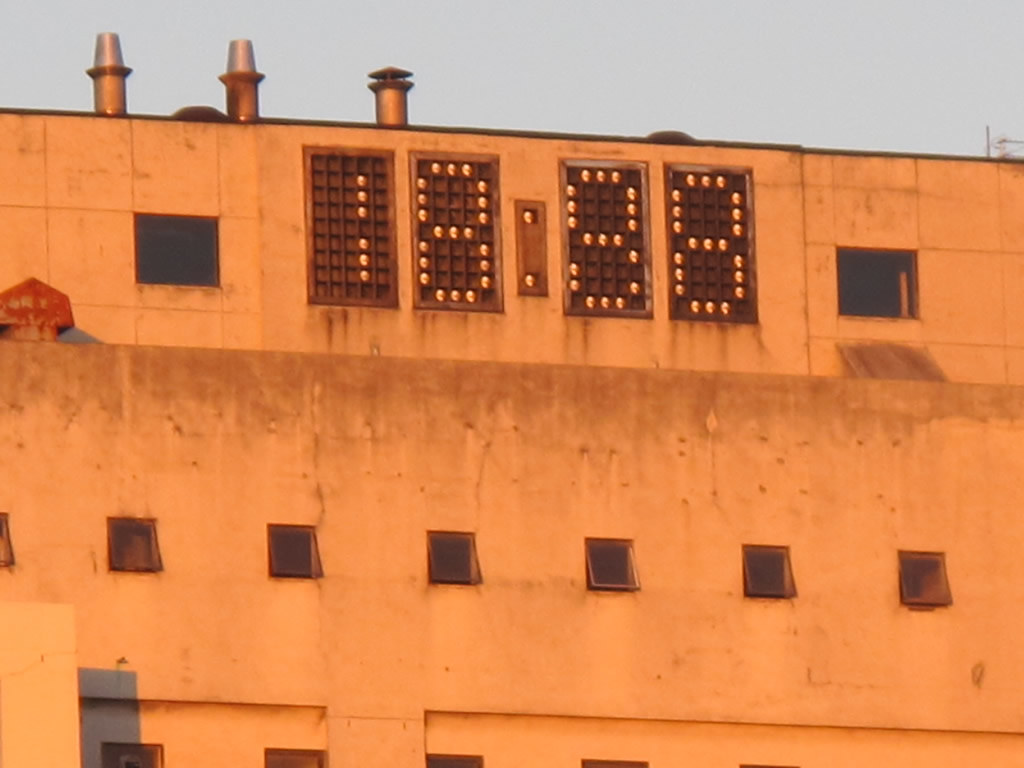This photograph showcases a close-up view of an older, tan-colored building, possibly a prison or some sort of institutional facility, indicated by its smaller windows on the lower levels and slightly larger windows above. Prominently displayed on the side of the building is an electronic display board resembling a scoreboard. The board reads "1888," which could potentially signify a countdown clock set to 18 minutes and 88 seconds, or possibly another function entirely, such as a time indicator in military format. The building also features several smokestacks on the roof, reinforcing the notion of an industrial or institutional setting.